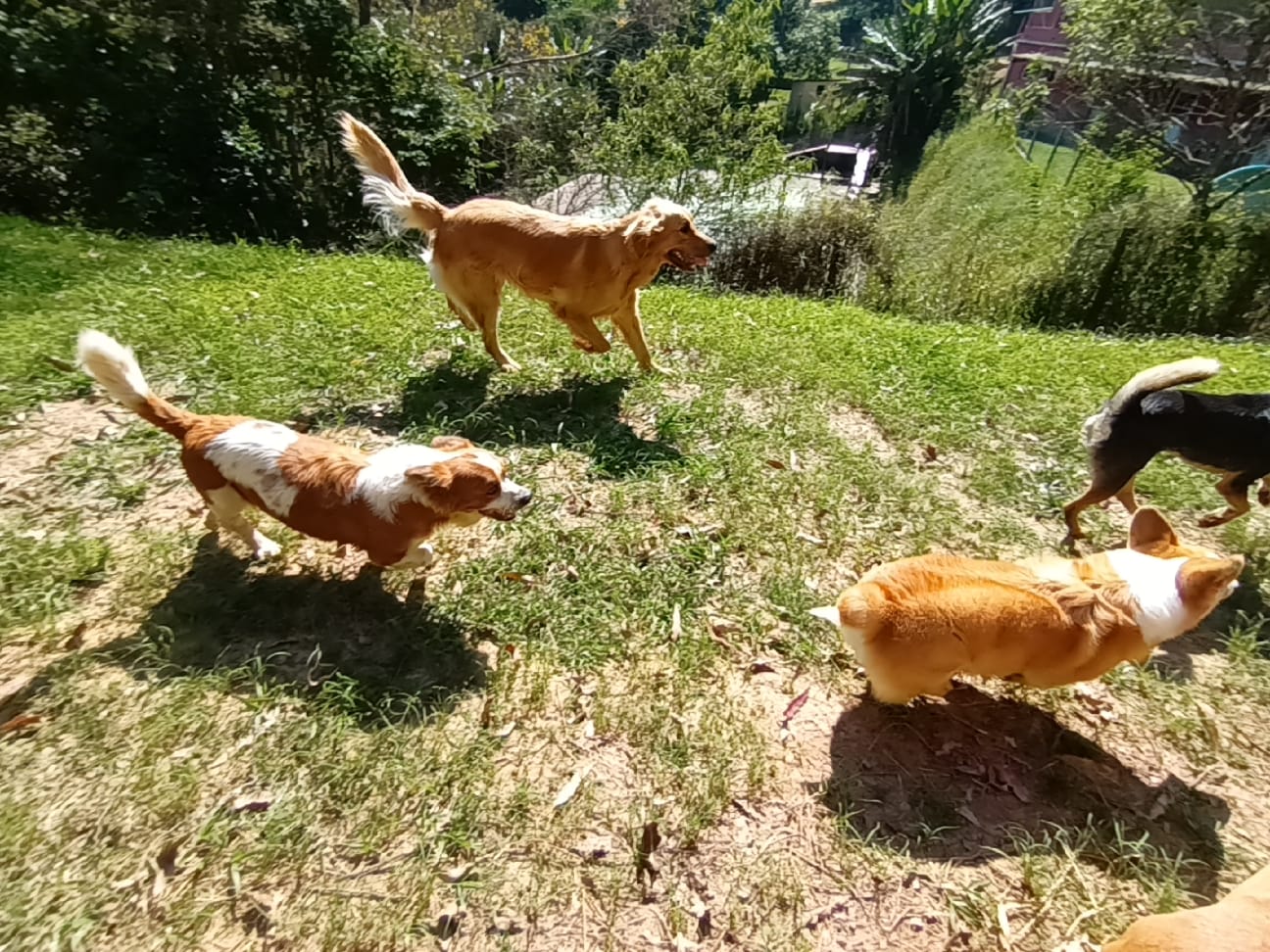This dynamic landscape photograph captures a lively scene of four dogs running from left to right across a grassy field, set against a forested backdrop. Dominating the foreground, a small golden brown corgi darts towards the right margin, its face obscured from view. Flanking it on the far right is a black dog with small fur and short brown legs, partially cropped by the photo's edge. Just behind them, a larger golden retriever bounds forward, its tongue playfully hanging out. Accompanying the retriever is a spaniel-type dog with distinctive brown and white markings. All the dogs, their tails held high, appear to be moving at a moderate pace. The image, taken from an elevated perspective, hints at a possible cliff or steep drop-off at the far side of the grassy area, suggesting the outskirts of a residential zone.